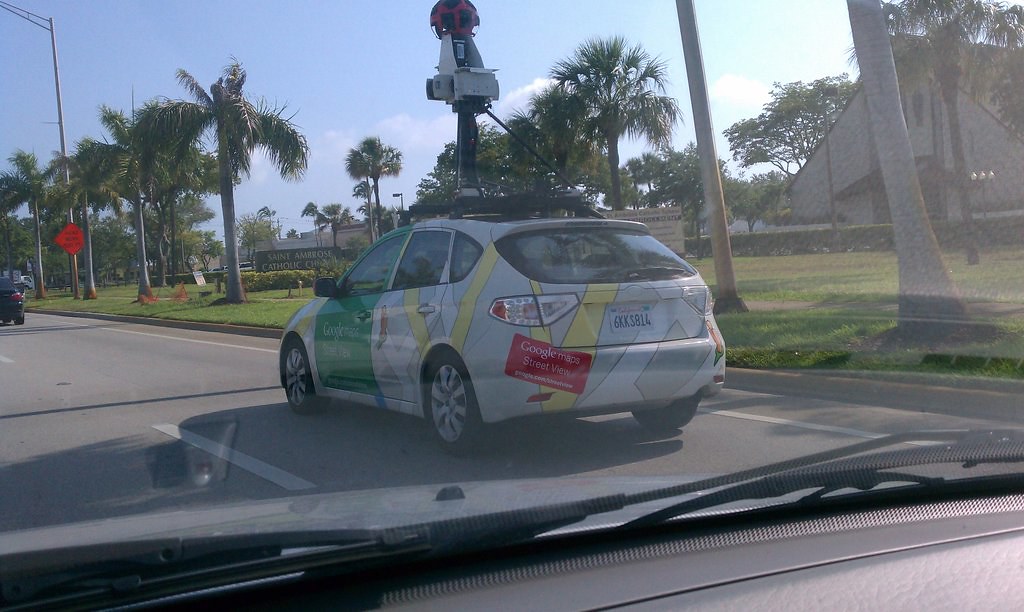In this overexposed horizontal photograph, taken from the driver's side of a car looking out through the windshield, the main focus is a small four-door white sedan identified as a Google Maps Street View vehicle. This car is seen driving ahead in the right lane of a two-lane highway, with a clearly visible large camera and GPS equipment mounted on its roof. The vehicle features a green door with white lettering and various map-related stickers overlaid on its white rear section. The photograph captures the scene from within a car, evident from the visible dashboard and windshield wipers. Surrounding the road is a tropical, park-like residential area, with numerous short, mature palm trees lining the grassy sides of the highway. In the background, there are street lights, hedges, and distant buildings, including a light-colored, almost triangular structure with dark brown doors and an awning. This detailed image captures the live mapping process in a lush, palm-dotted landscape.